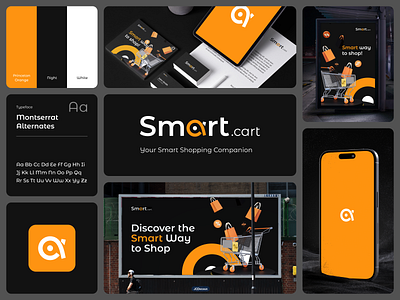The image is a detailed promotional layout for the "Smart.Cart," branded as "your smart shopping companion." The design is in a landscape orientation, composed of multiple segments arranged like a collage, highlighting various aspects of the product. 

The central section features a black background with the logo prominently displayed: "Smart.Cart," where the "A" in "Smart" is creatively designed to resemble a shopping cart in bold yellow. Below this logo, in small white text, is the tagline, "Your smart shopping companion."

To the top left, there's a vertical photograph with three color bars (yellow, black, and white) and some unreadable text. Directly below is an advertisement featuring white text on a black background, reading "Montserrat Alternates" with additional unreadable description beneath it.

The top center of the image showcases a picture of a mobile device, possibly a smartphone or tablet, displaying the Smart.Cart logo, surrounded by papers and objects, on a tabletop.

At the bottom center, a visual mimics a street sign board placed on a road. The background reveals a large wall, a lamppost, and a billboard that reads "Discover the Smart Way to Shop," featuring a shopping cart and padlocks. 

On the top right, there's an image of a bus stop advertisement sporting the same shopping cart icon and the tagline "Smart way to shop." Finally, the bottom right corner holds a photograph of a smartphone screen displaying the Smart.Cart logo within an orange background. 

The overall style is a blend of photographic realism and graphical design, making it visually engaging while effectively conveying the brand's message.